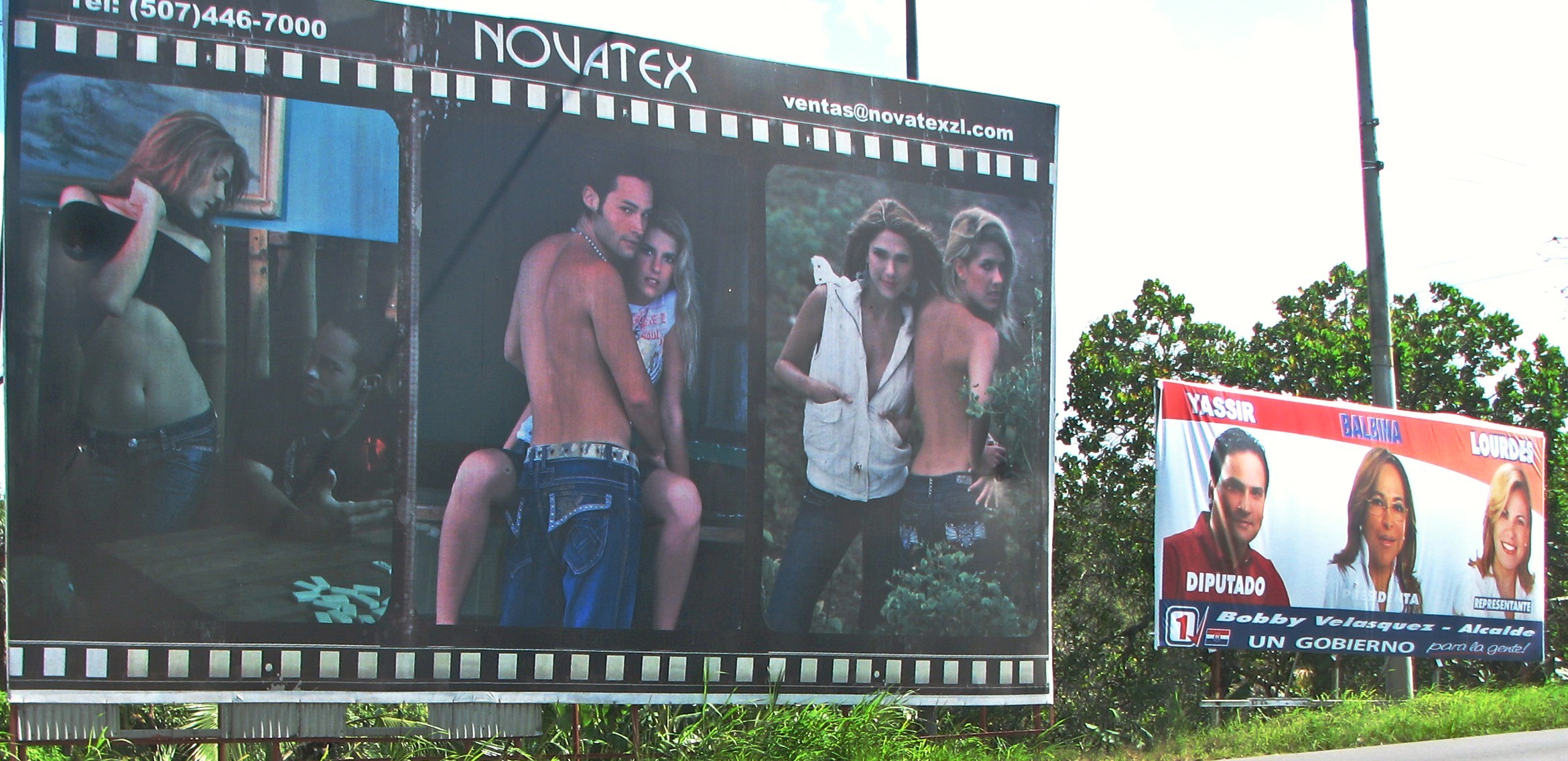The photograph captures a rural roadside scene featuring two prominent billboards set against a backdrop of green trees and dense vegetation. The left billboard, marked "Novatex" at the top with a contact number (507-446-7000) and an email (ventas at novatex.com), advertises a billboard sign company. Designed to resemble a film reel with perforated edges, it showcases three provocative images: a man at a table gazing at a sexy woman in a halter top and low-slung jeans, a shirtless man with a chain around his neck beside a sultry blonde woman on a counter, and two fashion models—one in a vest-style hoodie and blue jeans, the other bare-backed in jeans. To the right, a smaller, slightly sunken billboard presents three individuals—likely newscasters or political candidates—with a man labeled "Deputado" on the left, a dark-haired woman in the middle, and a blonde woman on the right.